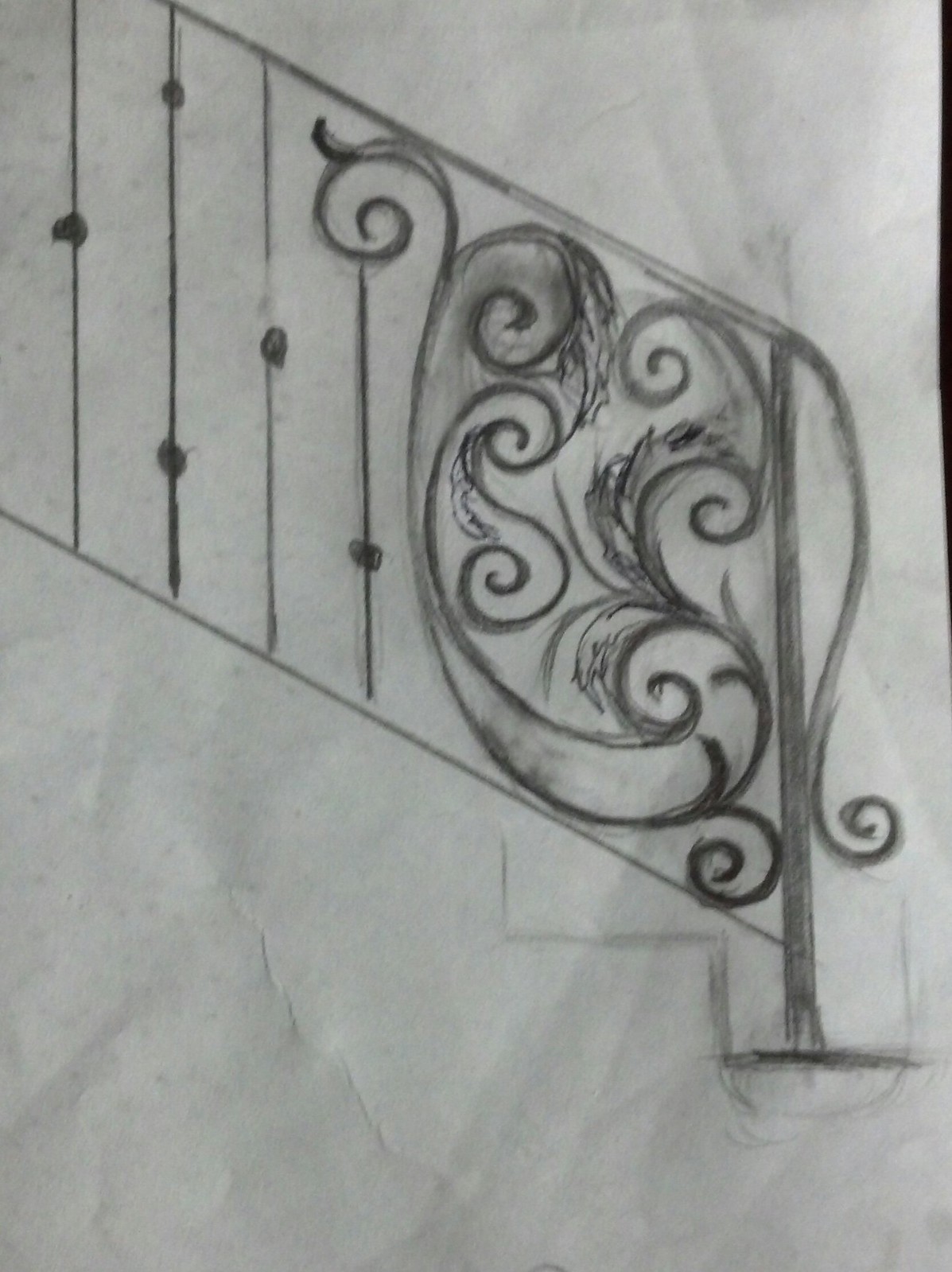The image depicts a detailed pencil drawing on a somewhat crinkled piece of white paper, illustrating an ornate staircase railing. The railing, likely a design concept, runs diagonally from the bottom right to the top left of the image. The lower section near the bottom steps features intricate scrollwork and twirls, reminiscent of old-fashioned wrought iron railings. The drawing includes several vertical bars adorned with circular knot-like decorations, resembling large buttons. The overall design is elaborate yet elegant, with the railing incorporating plant-like curves and dotted elements, indicative of thoughtful craftsmanship and revision. The staircase itself is only partially visible, with a few steps discernable at the lower right corner, enhancing the focus on the ornate handrail design.